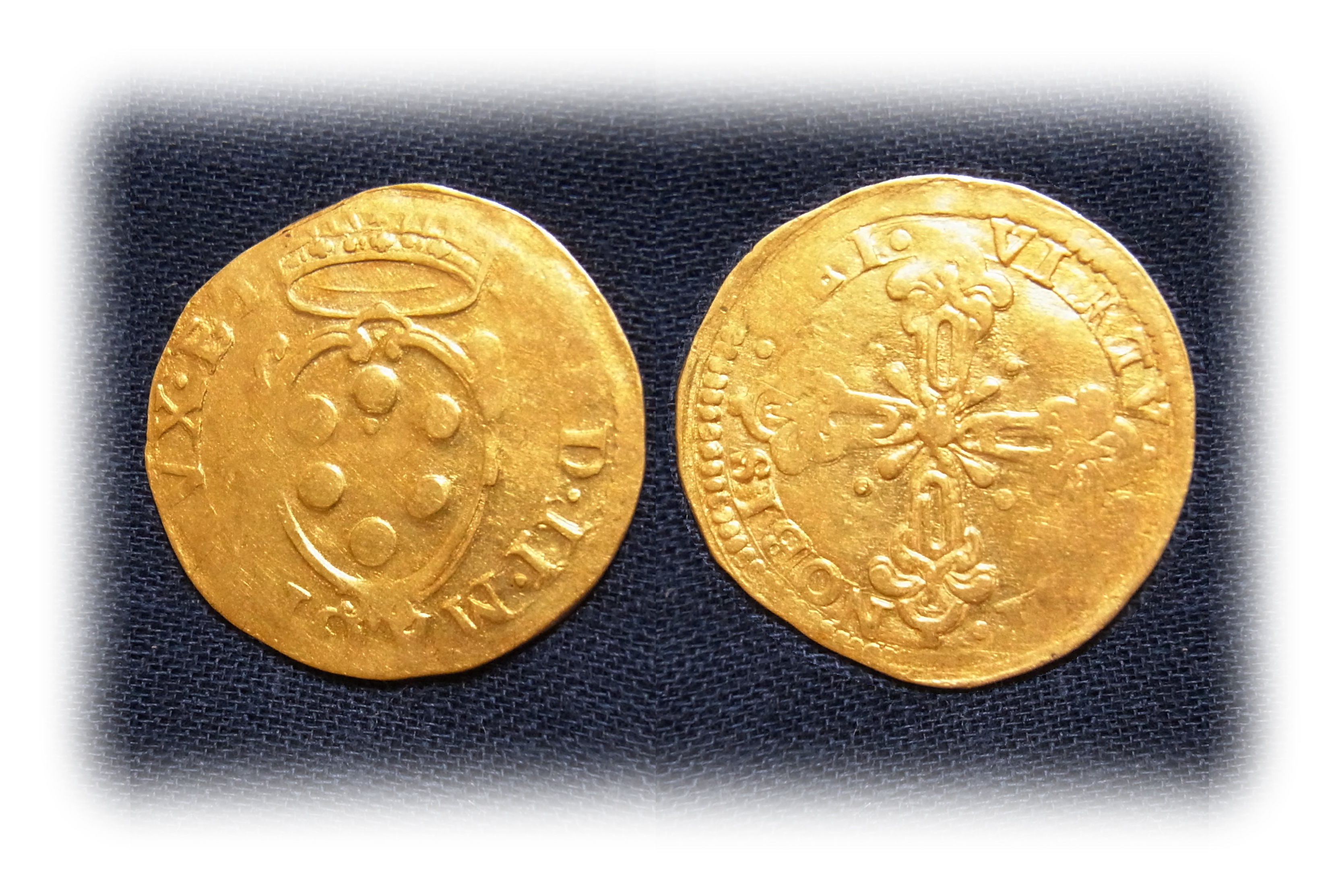This close-up image captures two gold-colored coins resting on a piece of black fabric. The left-side coin features a crown-like shape or perhaps an upside-down ring with intricate embroidery at the top. Beneath it, a main circle encloses six smaller circles arranged to form a triangular pattern. The outer edge holds faded inscriptions, suggesting it could be from the medieval era, or possibly Roman or Greek. The coin on the right boasts a cross-like design with frilled ends and additional frills radiating from the center. It appears to also have Latin writing and Roman numerals around the edge, which are quite worn. Both coins exhibit significant wear, particularly along their edges, and the imprints are partially faded, indicating their considerable age and historical value.